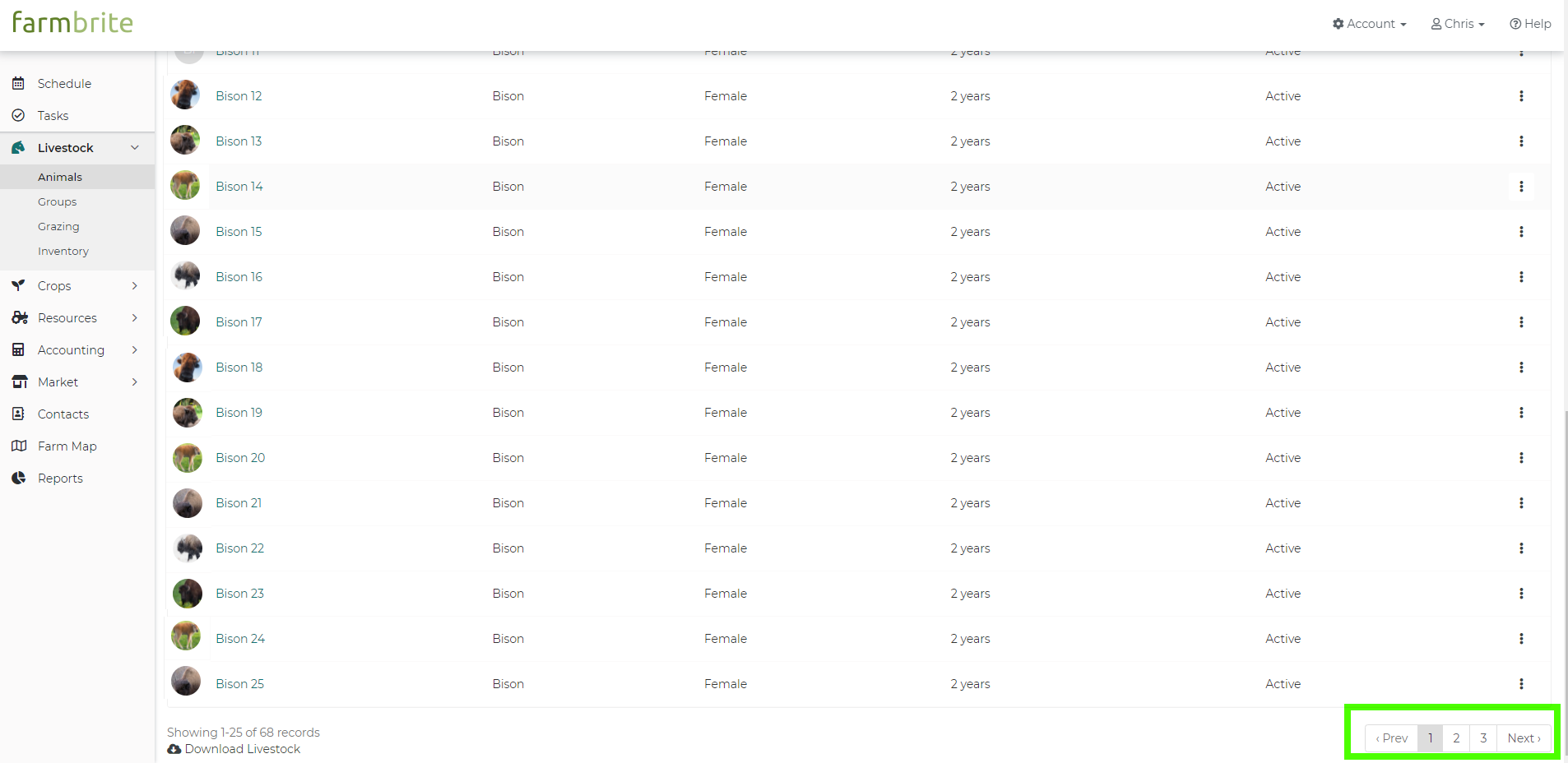The image depicts a detailed interface of a farming management software named "FarmBright." 

At the top left, there is a white background featuring the word "FarmBright" – "farm" is in dark green, and "bright" is in a lighter green, merged into a single word. On the top right, the navigation bar includes a drop-down menu with a gear icon labeled "Account," followed by a profile picture labeled "Chris." Adjacent to it, there is a circle with a question mark for "Help."

On the left-hand side, there is a vertical sidebar against a grayish background at the top, listing several sections: "Schedule," "Tasks," "Livestock," with an open drop-down menu that shows "Animals," "Groups," "Grazing," and "Inventory." Continuing on a white background, the sidebar includes "Crops," "Resources," "Accounting," "Market," "Contacts," "Farm Map," and "Reports."

On the right-hand panel, there is a table listing livestock details. The columns specify "Bison 12 through 25" on each line. The subsequent columns on each row mark the type ("Bison"), gender ("Female"), age ("Two years"), and status ("Active"). Each row ends with a vertical ellipsis (three dots).

Below the table, there is pagination information stating "Showing 1 of 25 of 68 results" alongside a "Download Livestock" button. On the right side, there are three page options encircled in green.

The comprehensive layout efficiently organizes farm management tasks, resources, and data for easy navigation and accessibility.